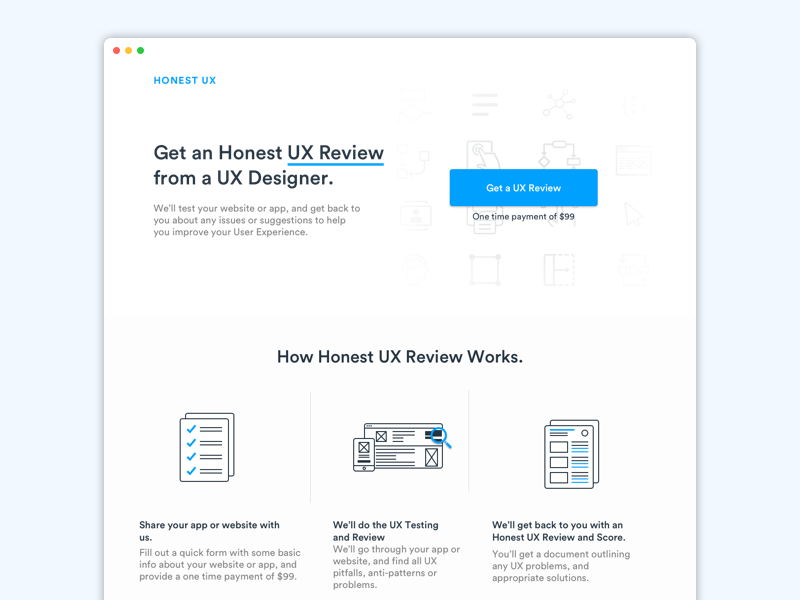The image showcases a website for a company named Honest UX. The company's name is displayed in the upper left-hand corner in a small, blue font. In the farthest upper left corner, there are three circles colored red, orange, and green. 

The central message on the website reads "Get an Honest UX review" with "UX review" underlined in blue. It continues with a promise: "From a UX designer. We'll test your website or app and get back to you about any issues or suggestions to help you improve your user experience."

On the right side, a light blue banner in a blue box proclaims "Get a UX review." Below this, in smaller text, it states "One-time payment of $99."

The website's background is not solid white but features images that include computers, a hand pressing a button, and a person holding a clipboard.

Towards the bottom section, the steps to receive an Honest UX review are laid out: 
1. "Share your app or website with us."
2. "We'll do the UX testing and review."
3. "We'll get back to you with an Honest UX review and score."

Each step is accompanied by detailed explanations.